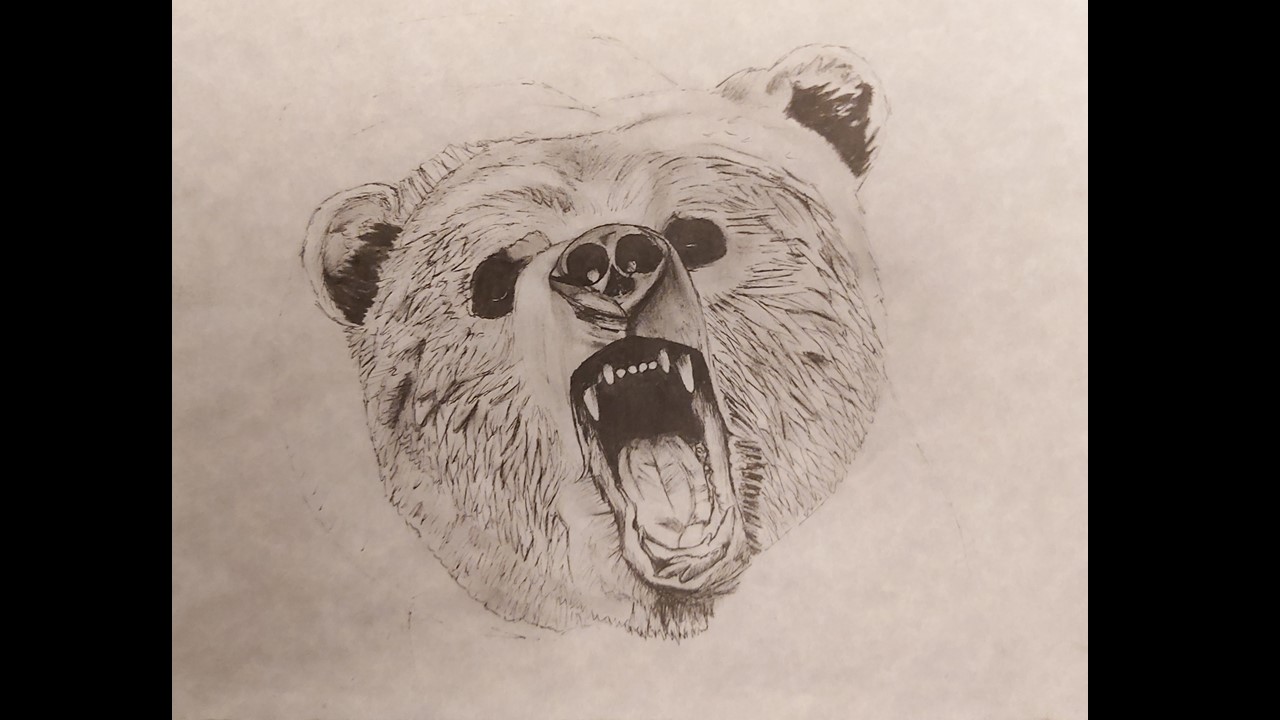A detailed black-and-white sketch on white paper showcases a powerful bear in a dynamic pose at the center of the composition. Created with meticulous pencil work, the bear's expressive posture features its head slightly tilted, drawing attention to its open mouth, which suggests a fierce roar rather than a gentle yawn. The artist has intricately detailed the thick fur, rendering a palpable sense of texture and depth. The bear's left ear, positioned towards the top right corner of the image, furthers the dynamic tension of the scene. Sharp teeth and a prominently displayed tongue at the bottom of the gaping maw enhance the raw, dramatic energy captured in this artwork.